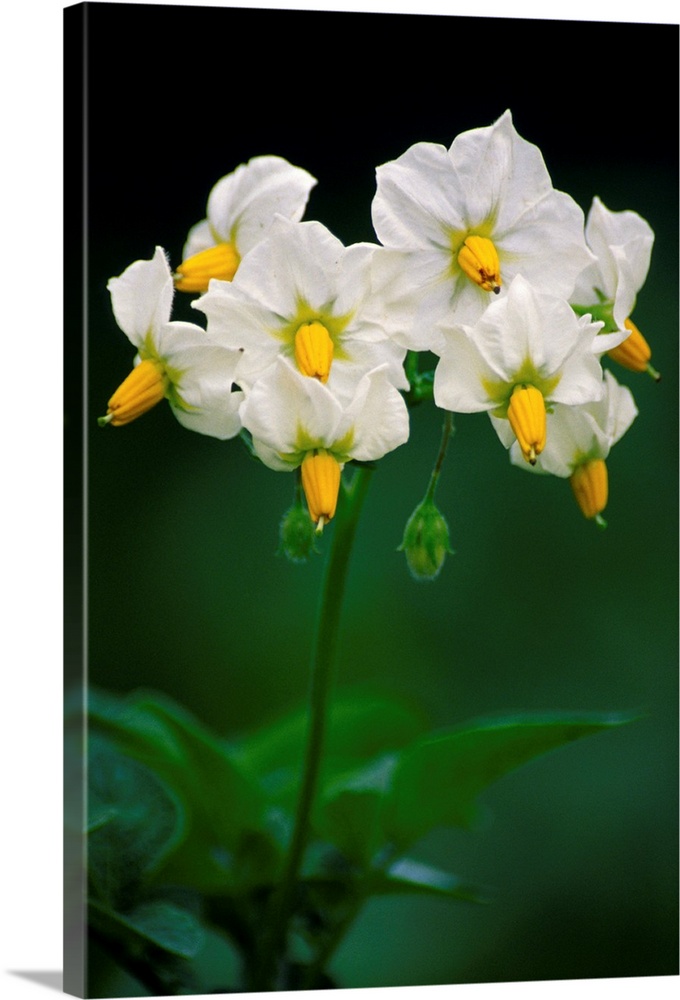This is a photograph stretched onto canvas, depicting a delicate white flower with a star-shaped arrangement of petals and a prominent yellow pistil at the center. The flower, which takes up the top half of the vertically oriented canvas, is the focal point with its detailed and soft-textured petals. Surrounding the yellow pistil is a subtle green hue. The stem extends downward, leading to green leaves that occupy the bottom portion in a bright, soft-focus bokeh style, adding a dreamy quality to the background. The fine details of a few unopened buds hang delicately beneath the flowers, blending into the blurred greenery. Captured in bright sunlight, this nature-inspired artwork showcases the ethereal beauty of the white star-like flower amid varying shades of green, all mounted on a frame designed to be hung on a wall.